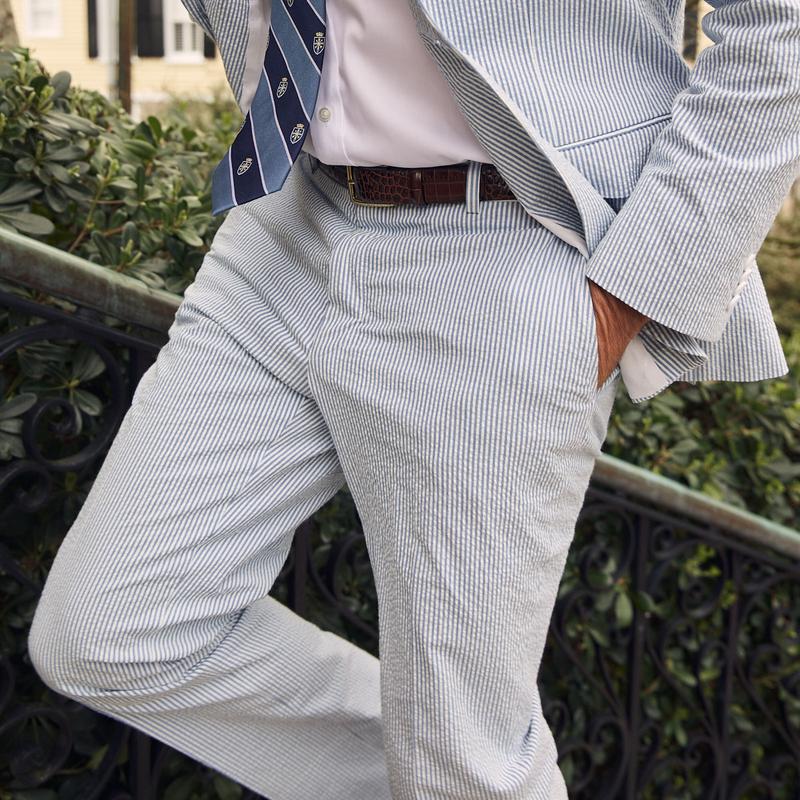In a modern, squared photograph, a Caucasian man is seen leaning against a metal railing, suggestive of an urban setting with hints of a city street visible in the top left corner. Green foliage adorns the background, partially obscured by the man's figure. The man is dressed in a matching blue and white pinstriped seersucker suit. His pants and jacket are both meticulously tailored with pinstripes, creating a sharp, stylish look highlighted by his dark blue and light blue diagonally striped tie. A pristine white dress shirt peeks out from under the suit, fastened with a black belt around his waist. He exudes casual confidence, standing with his right knee bent and his left hand tucked into his pants pocket. The photograph captures his lower half up to his chest, emphasizing his poised stance against the railing, with greenery and urban elements subtly framing the scene.